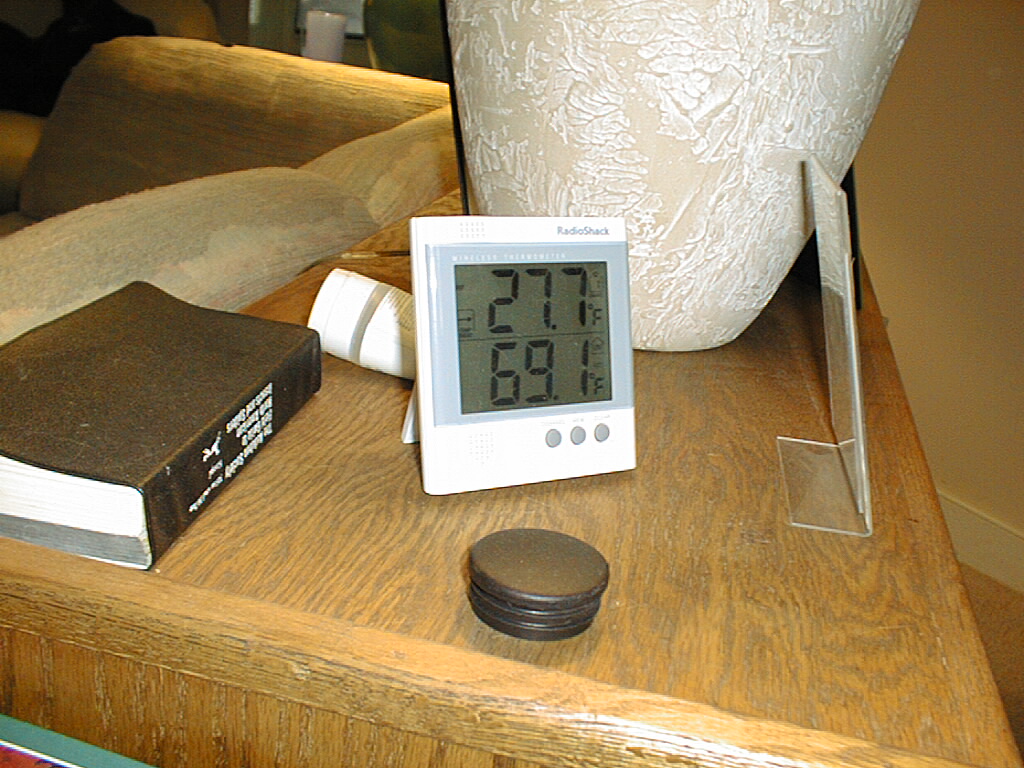In this landscape-oriented photograph, the primary focus is an aged wooden sofa table positioned behind a lightly worn, taupe-colored sofa with a rough texture, evocative of 1980s interior design. The table itself is light brown, reminiscent of oak, and carries an assortment of items each telling a small story of its own. 

Front and center on the table is the base of a ceramic lamp, distinguished by a pattern that appears impressed and highlighted with white paint, giving it a tan and white appearance that adds a touch of elegance to the setting. Nearby, there is a book lying face down, easily identifiable as an Audubon Society Bird Guide by its distinctive black, semi-vinyl plastic cover, known for featuring photographs and detailed information about various bird species.

Adjacent to these items sits a white plastic temperature readout device from Radio Shack, featuring a digital display and three light gray buttons below the screen. The display shows a temperature of 27.7°F on one part and 69.1°F on another, likely denoting outside and indoor temperatures, respectively. This perplexing readout is accompanied by what appears to be a large wooden stopper, around the size of a dollar coin, further adding to the eclectic mix on the table.

Lastly, a lotion bottle is situated behind the temperature device, next to a clear plastic display stand typically used for brochures, tying together this snapshot of a cozy living room environment, rich with details that hint at the personality and interests of its inhabitant.